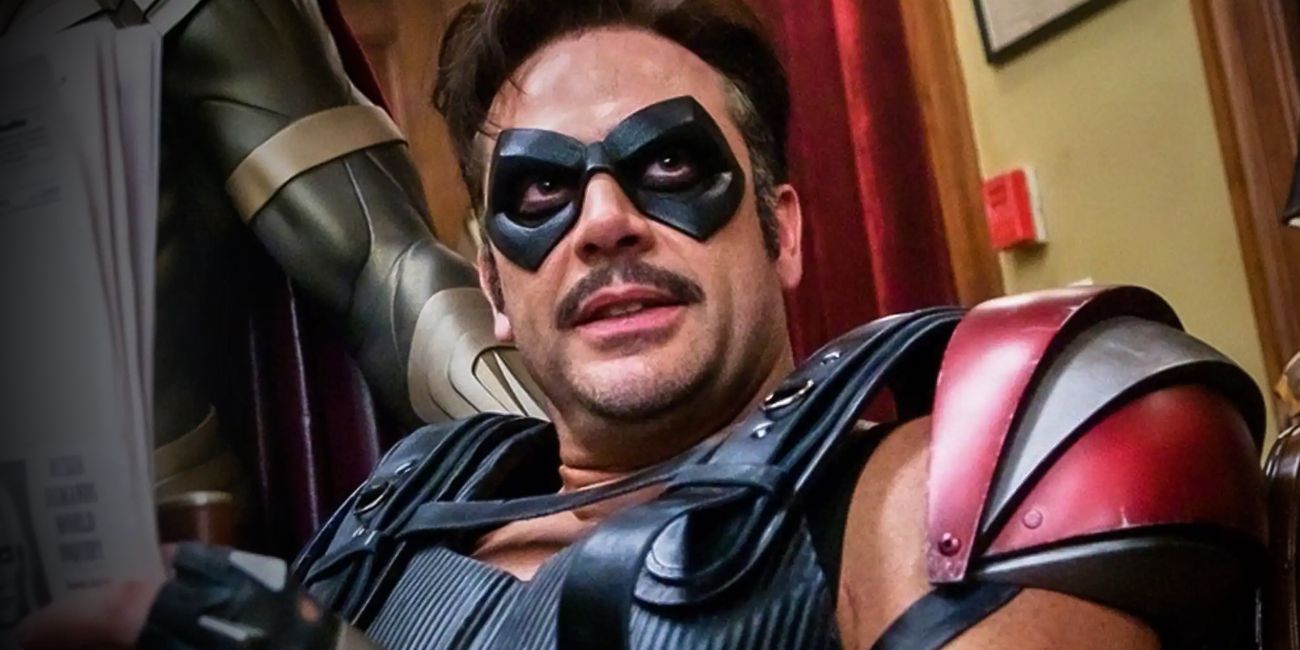The image depicts a scene from a superhero movie, likely "The Watchmen," featuring the actor Jeffrey Dean Morgan. The main character is a hefty man with a mustache and longer dark brown hair, partially held back by a headband. He is adorned in a distinctive black mask that covers only his eyes, resembling armor with a ridge over the nose, possibly made of metal or plastic. His foreboding eyes appear dark, most likely dark brown. His superhero costume is elaborate, featuring black straps over the shoulders, a black chest piece, and red and gray armor on the shoulders. Only his head and shoulders are visible, and his costume radiates a combination of black, gray, and red accents. To the left, another superhero, who might have a gray and gold or dark green suit, is partially visible with what seems to be a muscular, possibly robotic arm and a gray strap over the biceps. The background hints at an interior setting with a wall, a framed picture, and a red curtain, suggesting a detailed and immersive scene.